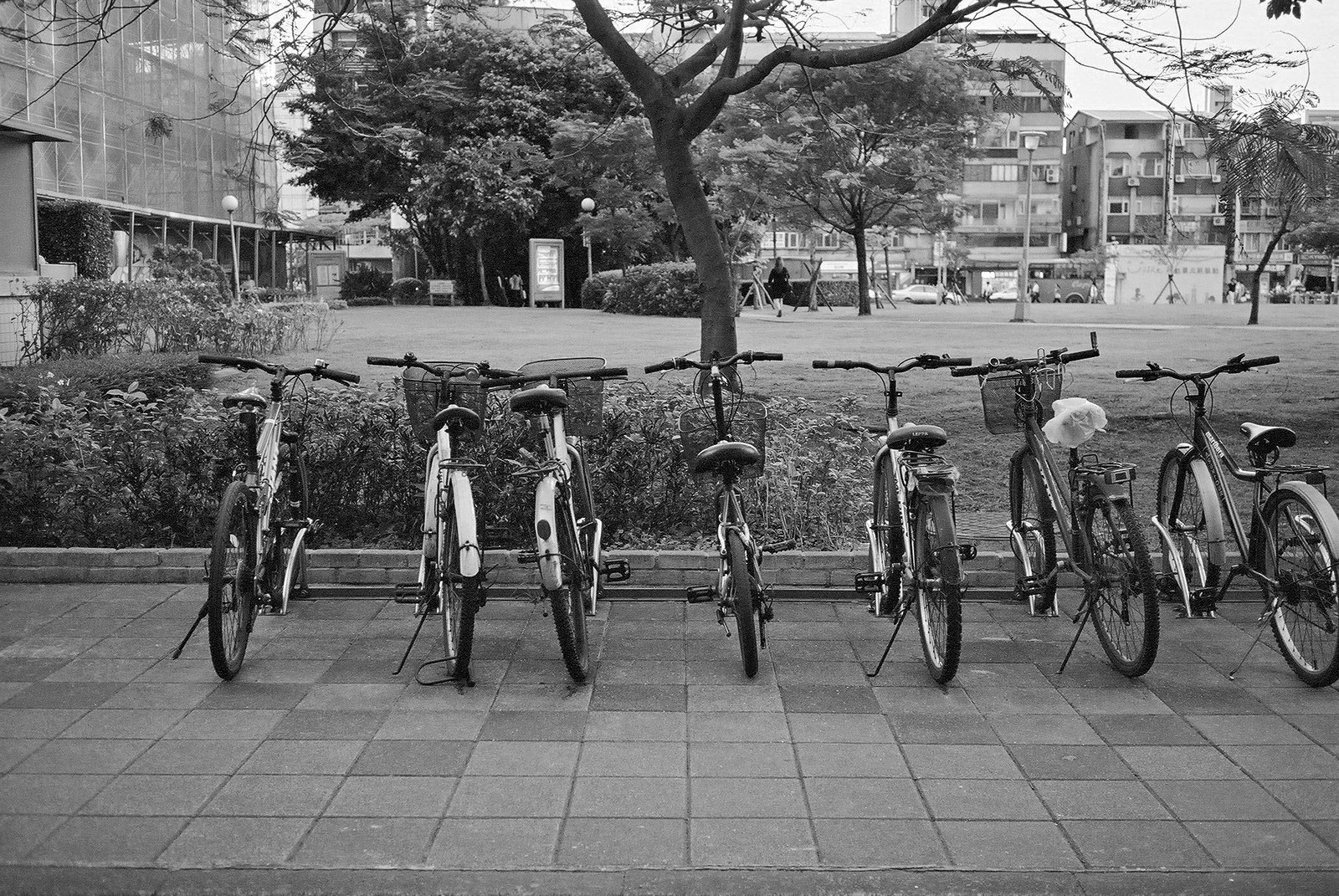In this detailed black and white photograph, seven bicycles are lined up side by side, propped up on kickstands and facing forward. The bikes rest on a dark grey paver walkway bordered by a low, two-brick-high wall. Their dark black wheels, chrome spokes, and black handles stand out, with the first two bikes on the left featuring a white tire trim, and the one on the right having a grey cover over its wheels. Several of the bikes have metal baskets attached.

Behind the row of bicycles, there are two-foot-high bushes leading into a park-like area dotted with leafless tree branches and a larger tree with some leaves. Further out, light poles are visible, adding character to the serene landscape. To the left of the image, there's a building with many windows, which appears to be under construction, evidenced by scaffolding and mesh coverings. In the background, beyond this park area and across a roadway, additional buildings and parked cars are visible, along with a bus. The photograph captures a tranquil yet dynamic urban setting, possibly a campus, under a light grey sky.